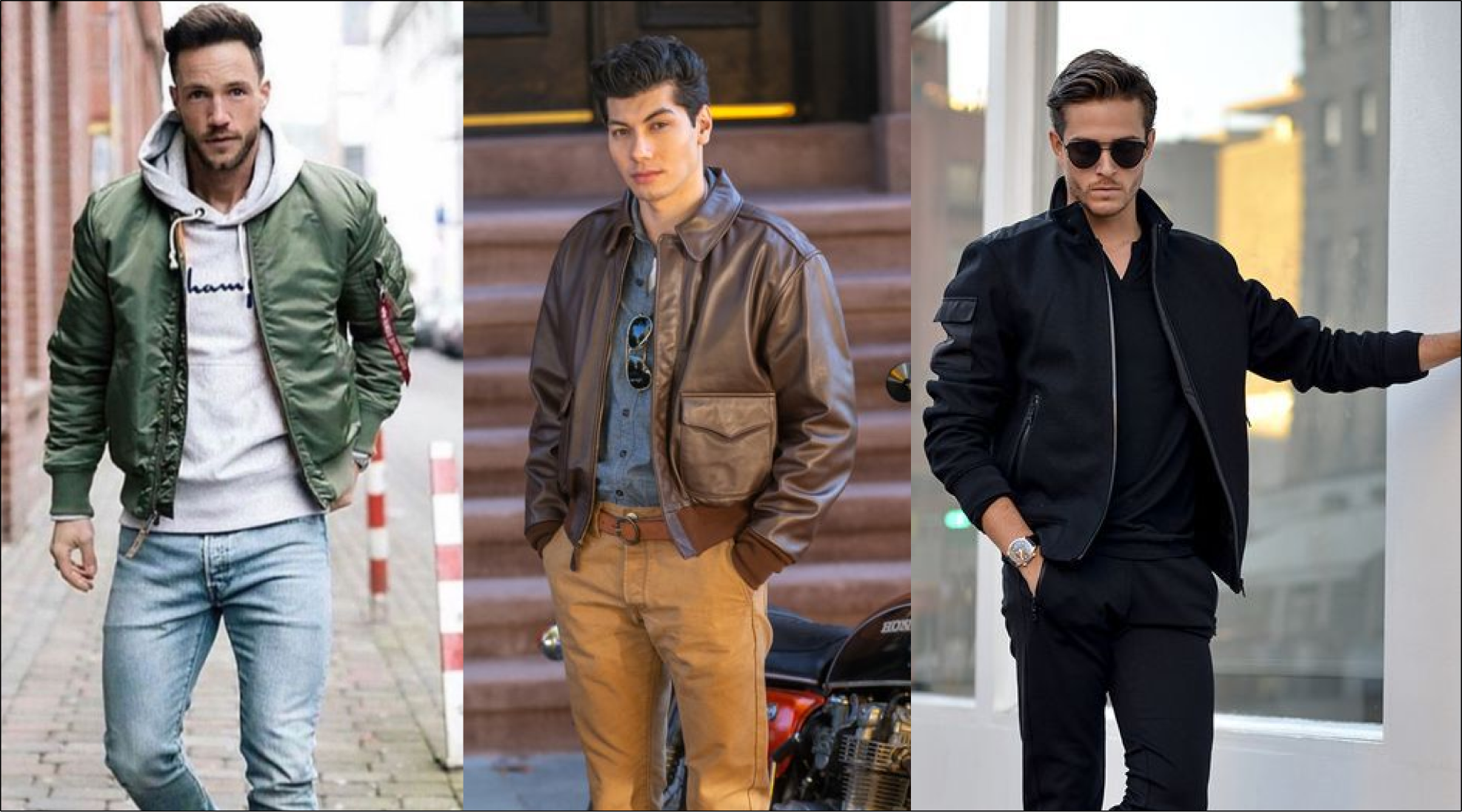The image presents a collage of three vertical photographs, each capturing a stylishly dressed man posing for what appears to be a fashion shoot. The first man, situated on the left, stands on a concrete sidewalk with an orange-striped pole and a brick building in the background. He dons a layered look with a gray Champion-branded hoodie under a green, open jacket, complemented by blue jeans and dark blonde to light brown hair. He has a beard and mustache and looks directly at the camera.

The middle photo features a man with brown hair and sunglasses tucked into his blue button-up shirt. He sports a sleek brown leather jacket along with tan pants and a matching brown belt. Behind him, a set of steps and two doors, along with what appears to be a motorcycle, contribute to an urban backdrop. He too looks straight into the camera.

The rightmost image showcases a man in black attire, including a black jacket over an unzipped black polo shirt, and black pants. He accessorizes with black sunglasses and a watch on his right wrist, his hand in his pocket. He poses with his left hand slightly extended and stands in front of a large window, immersed in what seems to be a cityscape. Each man exudes a distinct style, emphasizing a curated display of fashionable outfits and poses.